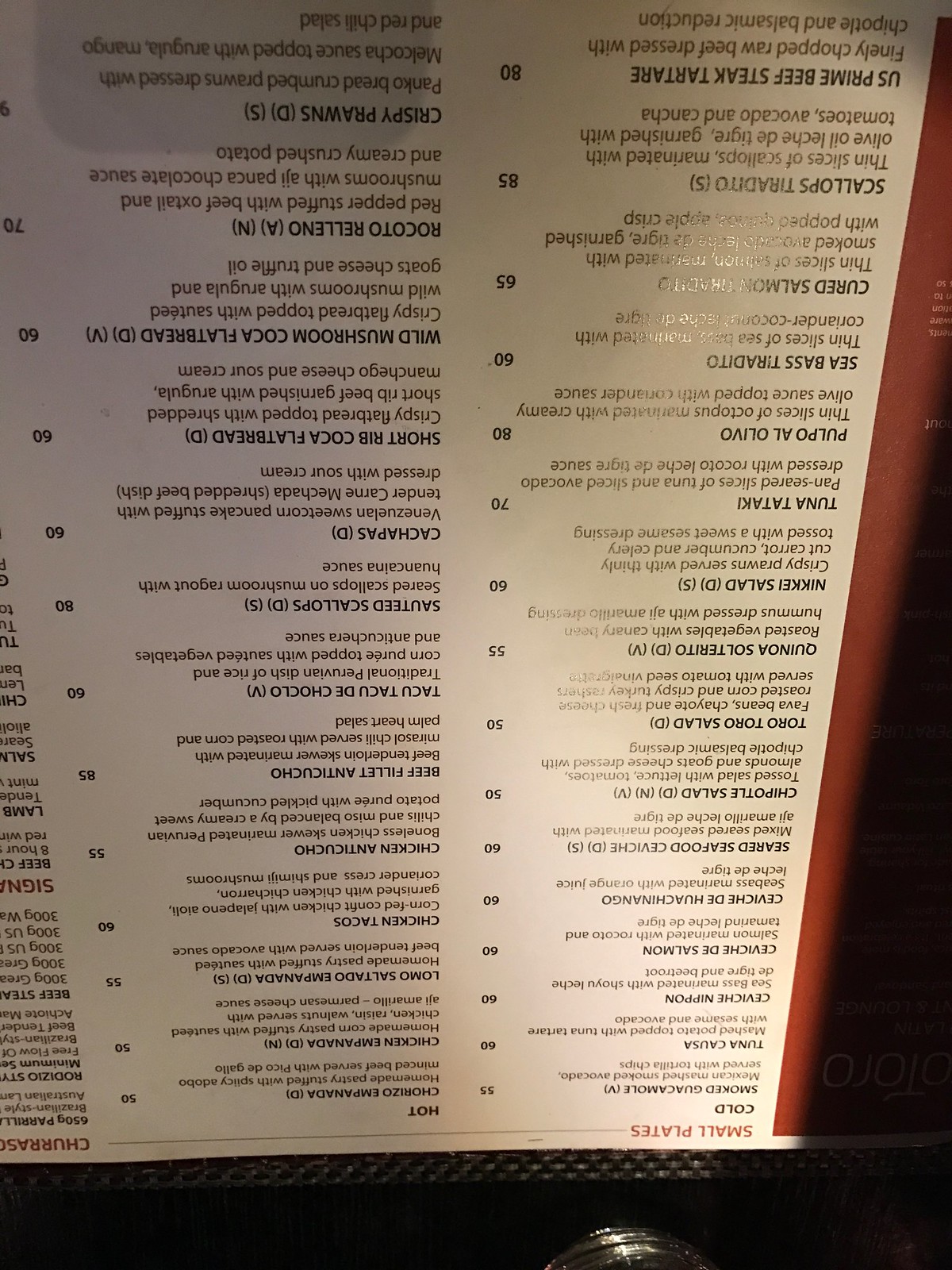This color photograph captures an upside-down view of a restaurant menu, making it a challenge to decipher the items listed. The menu features an array of sophisticated offerings, starting with the "Small Plates" section. Highlighted dishes include Tuna Tartare priced at $70 and U.S. Prime Beef Steak Tartare at $80, indicating the restaurant's upscale nature. Additionally, the menu presents Crispy Prawns and Wild Mushroom & Cocoa Flatbread among its selections. 

Further, the menu offers both cold and hot plates. Under the hot food category, Chicken Tacos and an intriguing Chicken & Artichoke dish are listed. The presence of Short Ribs reflects a level of culinary delicacy typically found in high-end steakhouses. Each section showcases a different aspect of the restaurant’s diverse and gourmet cuisine, with the prices underscoring its exclusivity and premium dining experience.